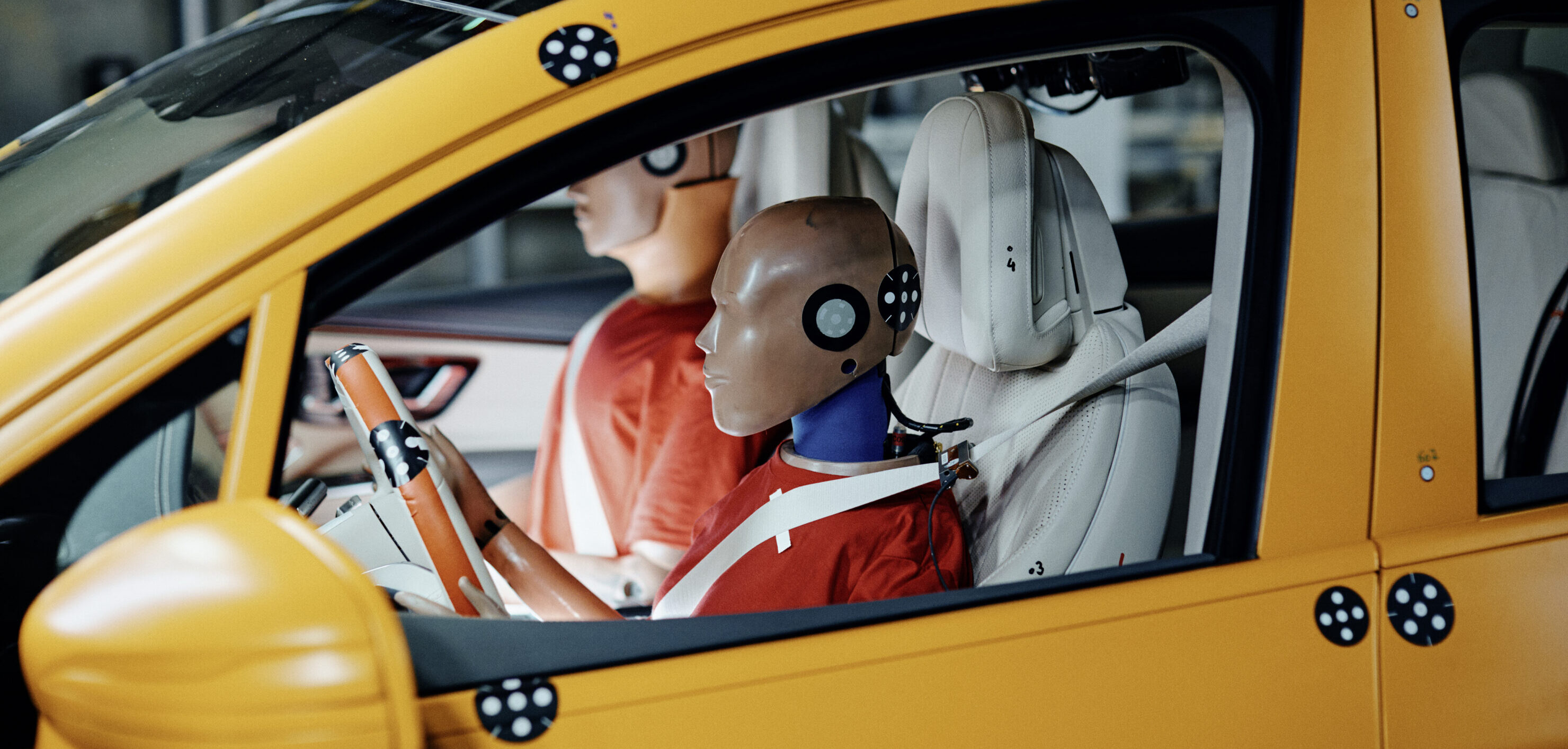The photograph depicts a pair of crash test dummies seated in the front of a bright yellow vehicle, resembling a taxi cab, with tan leather interiors. Both dummies are strapped in with white seat belts and are dressed in orange T-shirts. The dummy in the driver's seat grips the steering wheel with both hands, while the passenger dummy rests its hands on its lap. Each dummy has specific sensors, including black headgear dotted with white circles and black circular markers with white centers near their ear areas. The vehicle's exterior is also adorned with black stickers featuring five white dots, likely used for positioning in crash testing scenarios. The driver's side window is open, providing a clear view into the meticulously prepared scene for an impending crash test, with no occupants visible in the back seat.